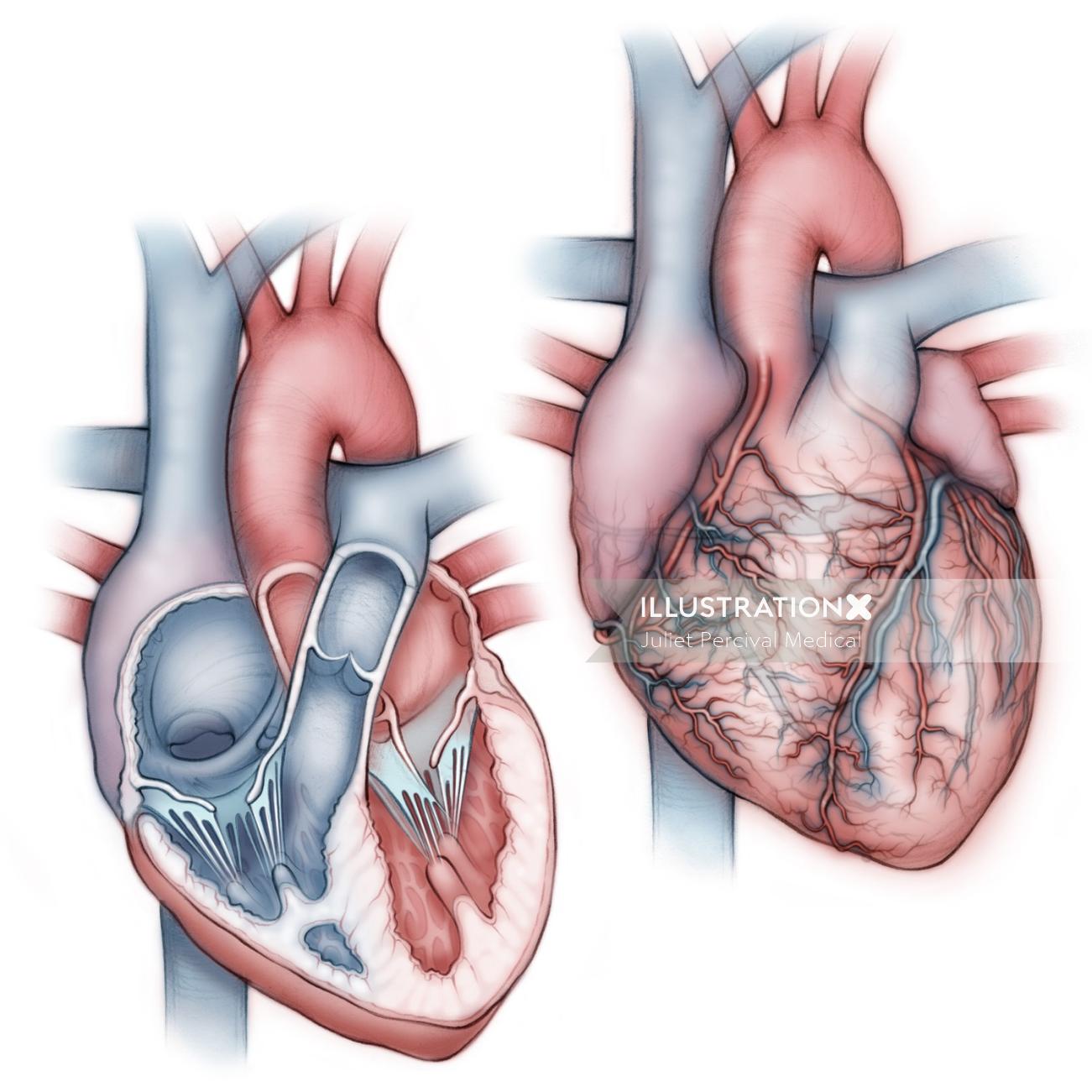This illustration showcases two depictions of a heart. On the right, the exterior view of the heart is detailed with a complex network of veins and arteries, rendered in vibrant blue and red, signifying blood flow. The left side presents a cutaway view, uncovering the internal structure. Both images are rich in anatomical detail, showing various veins, capillaries, and nerves in red and blue, aligned in intricate patterns. The background is stark white, enhancing the clarity of the illustration. Hovering in a semi-transparent white box, textual elements in white capital letters read, "Illustration X Julie Percival Medical."